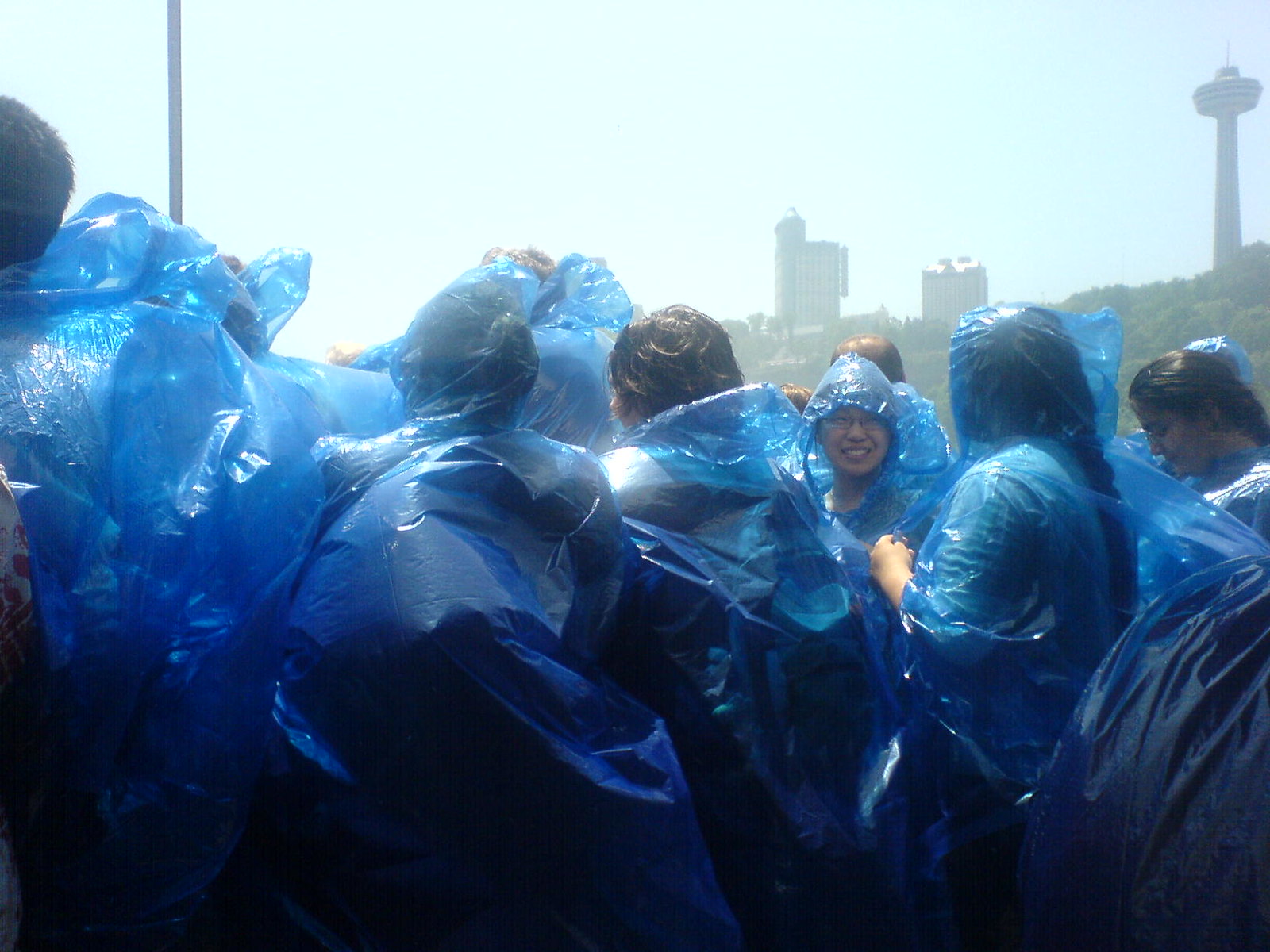A group of people stands outdoors in the rain, all clad in bright blue, thin transparent ponchos that flutter in the wind. Some of the ponchos have hoods up, covering wet hair, while others have their backs turned towards the camera. One woman with glasses faces the camera, her face lit by a half-smile. The sky above is a light blue-gray with hints of white clouds, adding to the hazy mist in the air, possibly from nearby rain or a waterfall. The background showcases a landscape of low bushes and hills, contrasted by three large buildings: a tall one with a circular window tower on the left, a shorter rectangular building to its right, and a structure resembling the Space Needle with a cylindrical base and a thick, rounded top.